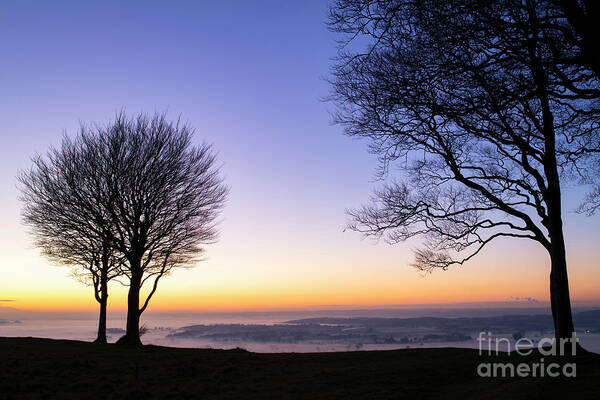This landscape photograph, taken in wide-angle view and in a color, representational realism style, captures a serene coastal area at either sunrise or sunset. Dominating the right side of the foreground is a tall, leafless tree with naked branches silhouetted against the vibrant sky. To the left, two smaller leafless trees with similarly wide canopies stand, contributing to the stark, barren beauty of the scene. These trees are rooted in a flat, possibly snow-covered or coastal sand surface that extends towards the horizon. The landscape between the trees and the horizon features rocky atolls, adding texture to the expansive white mass that could be interpreted as either snow or sea ice with low, transparent ocean waves gently coming ashore, their color a subtle light purple. At the horizon, a glowing orange band signifies the rising or setting sun, which casts the foreground into shadow. The sky above the horizon shifts from a light yellow to a gradient of blue that intensifies in darkness towards the top of the photograph. A subtle watermark reading "Fine Art America" is located in the bottom right corner, with a 50% white tint enhancing its visibility.